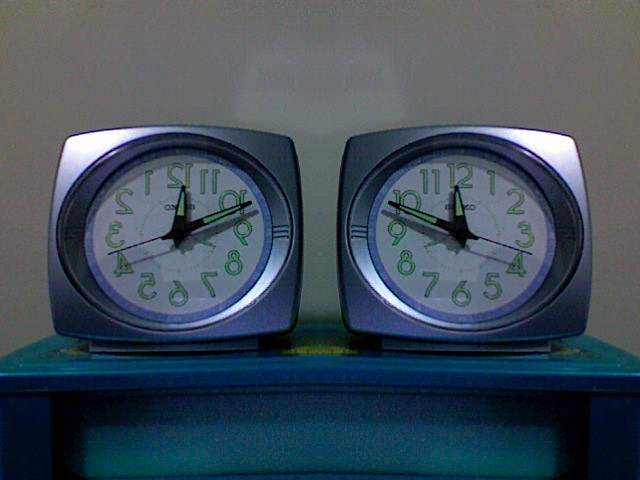The photograph captures two nearly identical square clocks, each housed within a simulated metallic silver plastic case. These clocks have white faces with lime green numbers and black and green hands, set against the backdrop of a white wall. Both clocks are positioned side by side on top of a blue table, which features a middle section that appears to be made of glass, reflecting light from the room.

The unique aspect of these clocks is that while the one on the right follows the traditional 1 to 12 arrangement in a clockwise manner, the clock on the left features a mirrored arrangement, with the numbers running counterclockwise. Despite this mirrored configuration, both clocks display the time as 12:10.

The focal point of the image accentuates the duality and mirrored nature of the clocks, contrasting the conventional setup with a quirky, reversed version. The table supporting the clocks is partly visible, showing some of its legs, but its drawer configuration remains undetermined due to the limited view. The overall setting suggests an indoor environment, possibly a house, with the image capturing the clocks from the perspective of someone standing in front of them.